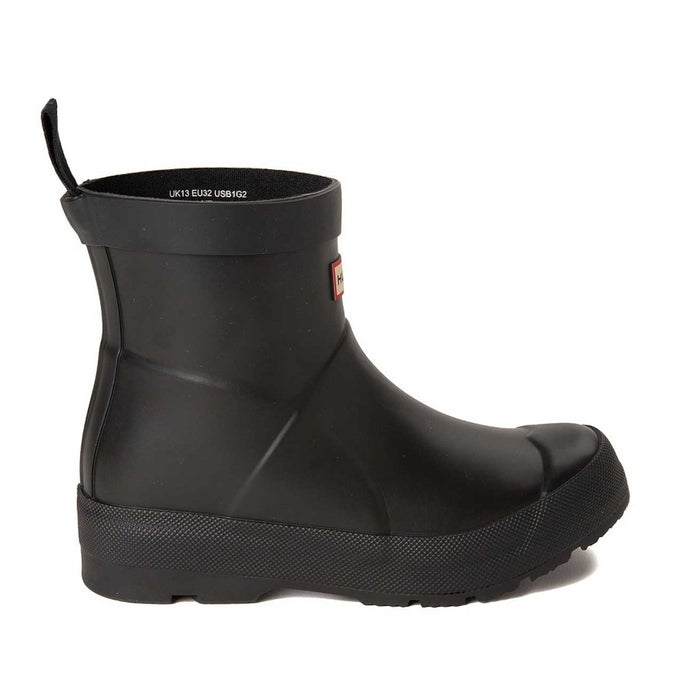This image captures a close-up view of a single black boot, which resembles a short ankle boot, slightly rising above the ankle. The boot is primarily black with a smooth texture, possibly made of leather or faux leather, accented by subtle thin black lines adding a touch of texture. Along the base of the boot runs a black textured band featuring very tiny diamond shapes, giving it a rugged appearance. 

The sole appears to be made of rubber, adding to the practical, utilitarian design of the boot. At the back and top of the boot, there is a functional black fabric loop, designed for effortless wearing by hooking a finger through it. The inner top band of the boot is adorned with white lettering indicating size labels: UK13, EU32, and USB1G2.

Towards the front, near the top of the boot, there is a distinctive tan label boxed in red with partial black lettering visible, hinting at the brand name, though the complete name can't be discerned—only an 'H' is visible. This label likely indicates the brand, contributing to the overall design detail of the boot.